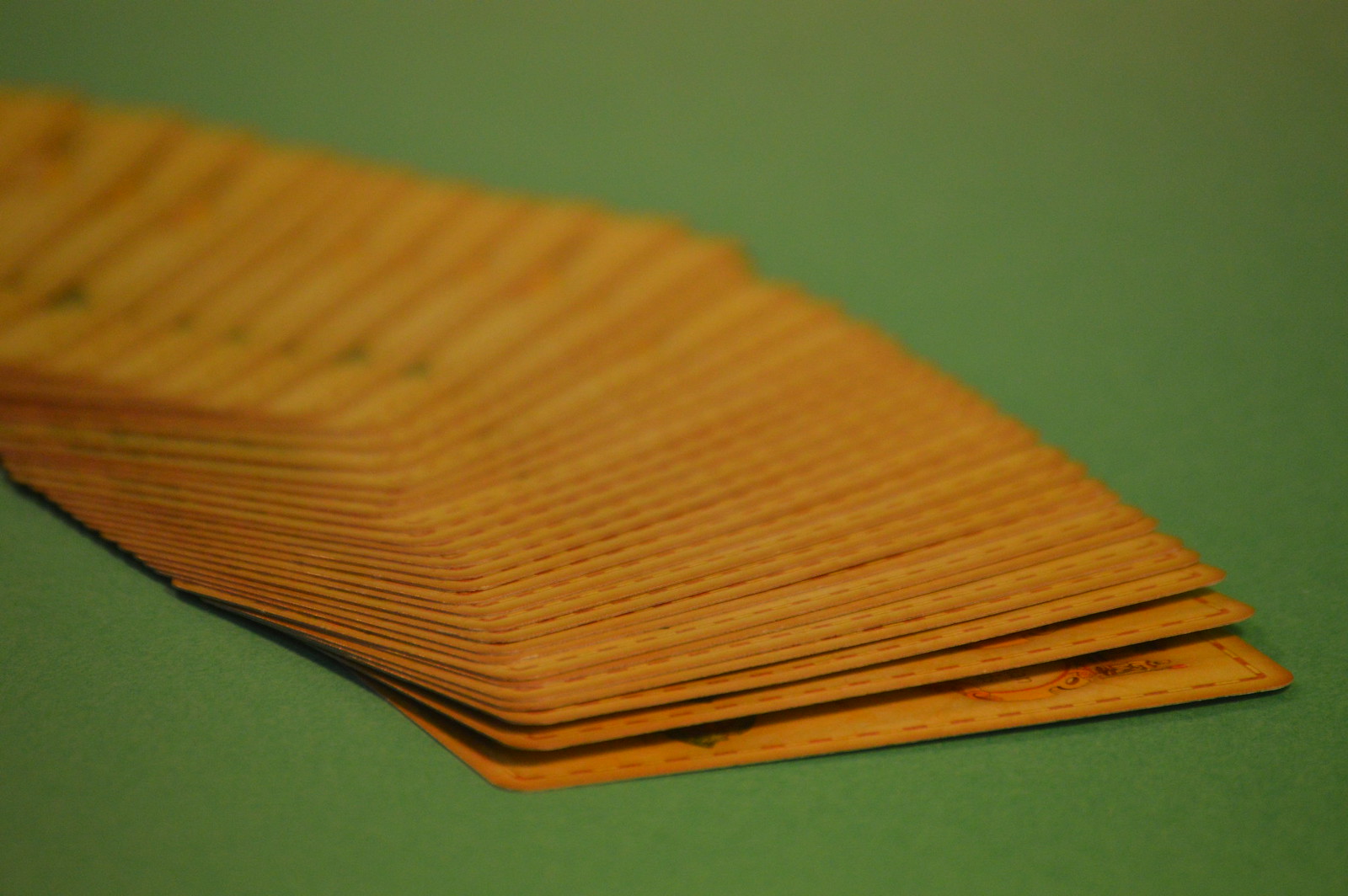A color image, seemingly AI-generated and significantly blurry, features a spread of aged playing cards against a green backdrop. The playing cards, originally white, now exhibit a yellowed, antiquated hue, indicative of extensive use and age. Each card is bordered with a red dashed line, and their corners are noticeably bent and worn. The cards, amounting to roughly 30 to 40—or possibly even the full deck of 52—are splayed out in a disorganized fashion on the green surface, which is likely not carpet despite its appearance. The blurriness obscures any specific details or lettering on the cards, but their timeworn and musty condition is evident.